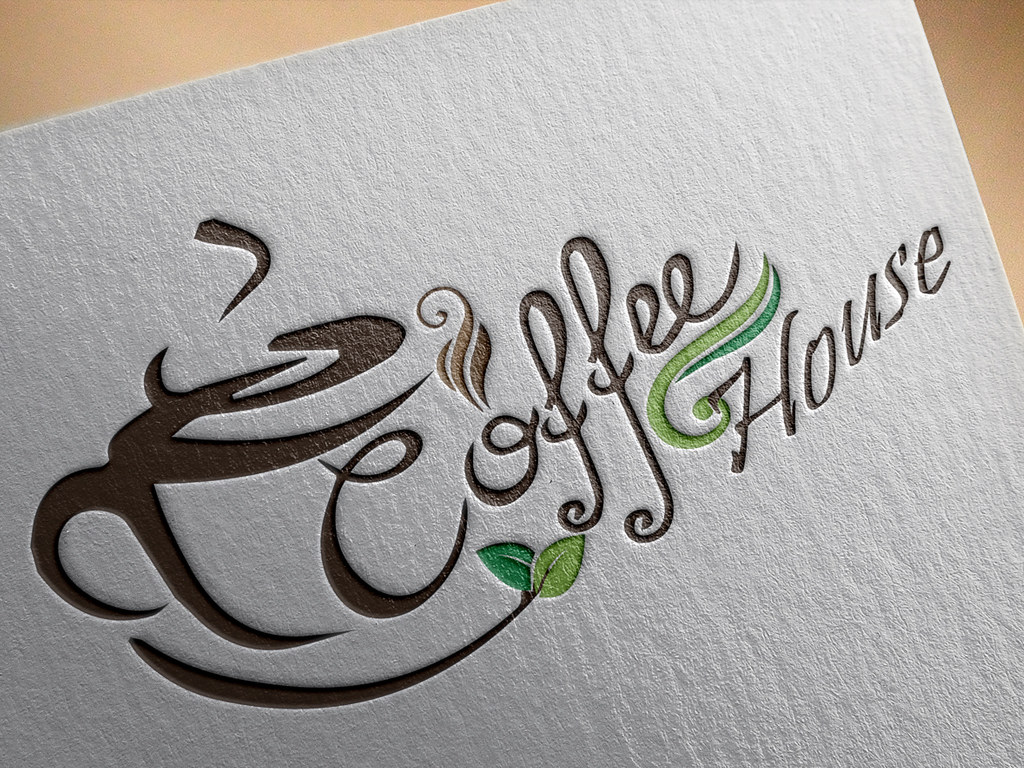The photograph showcases a textured piece of thick stock paper positioned at an angle on a tan-colored table. The paper has an elegant, embossed design featuring the words "coffee house" in a dark brown, script-type font, with an uppercase "H" and the rest of the letters in lowercase. Central to the design, an illustration creatively integrates elements of a coffee cup within the text: the letter "C" is stylized as a cup complete with a handle and brown wisps of steam rising from it, similar to the steam depicted coming out of the "O" in "coffee." Surrounding the text, a green swirl motif wraps around the word "house" and extends under "coffee," connecting to a delicate branch with two small green leaves, adding an organic touch. The white background enhances the visual appeal of the design, which likely serves as a napkin or an advertisement within a coffee house setting.